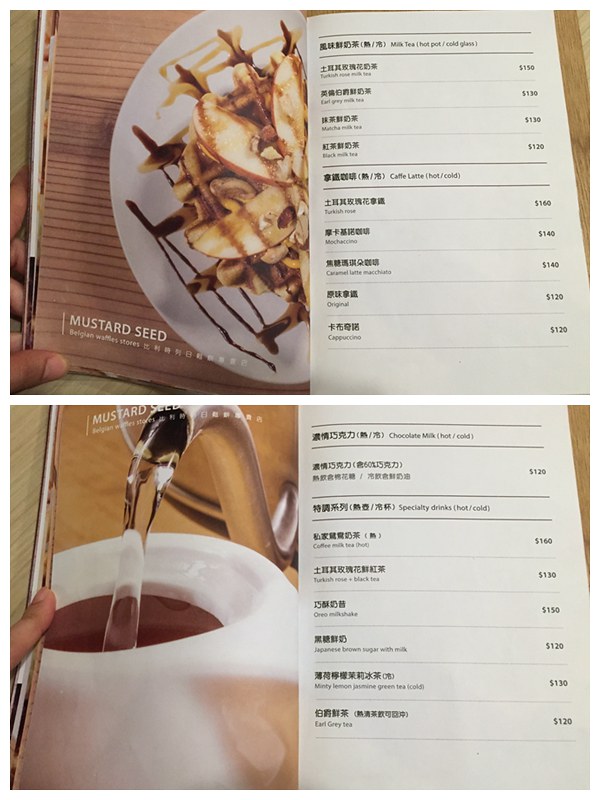The image contains two color photographs, stacked vertically, with a thin white border separating them. Each photograph displays an open cookbook. In both images, the left-hand page features a photograph, while the right-hand page contains text in a foreign language, listing items in a markdown format with prices aligned in the right-hand column.

In the top photograph, the left page showcases a dish labeled as "mustard seed." The image reveals a white plate with several apples, drizzled with what appears to be hot fudge or caramel, suggesting a dessert. However, despite the name "mustard seed," the visual elements imply a sweet treat rather than a savory dish.

The lower photograph on the left side of the cookbook depicts a white coffee cup being filled with clear water from a pewter-like pitcher. The inside rim of the cup, or potentially the liquid it contains, is brown. Human fingers are visible on both sides of each photograph, indicating that the book is being held open.